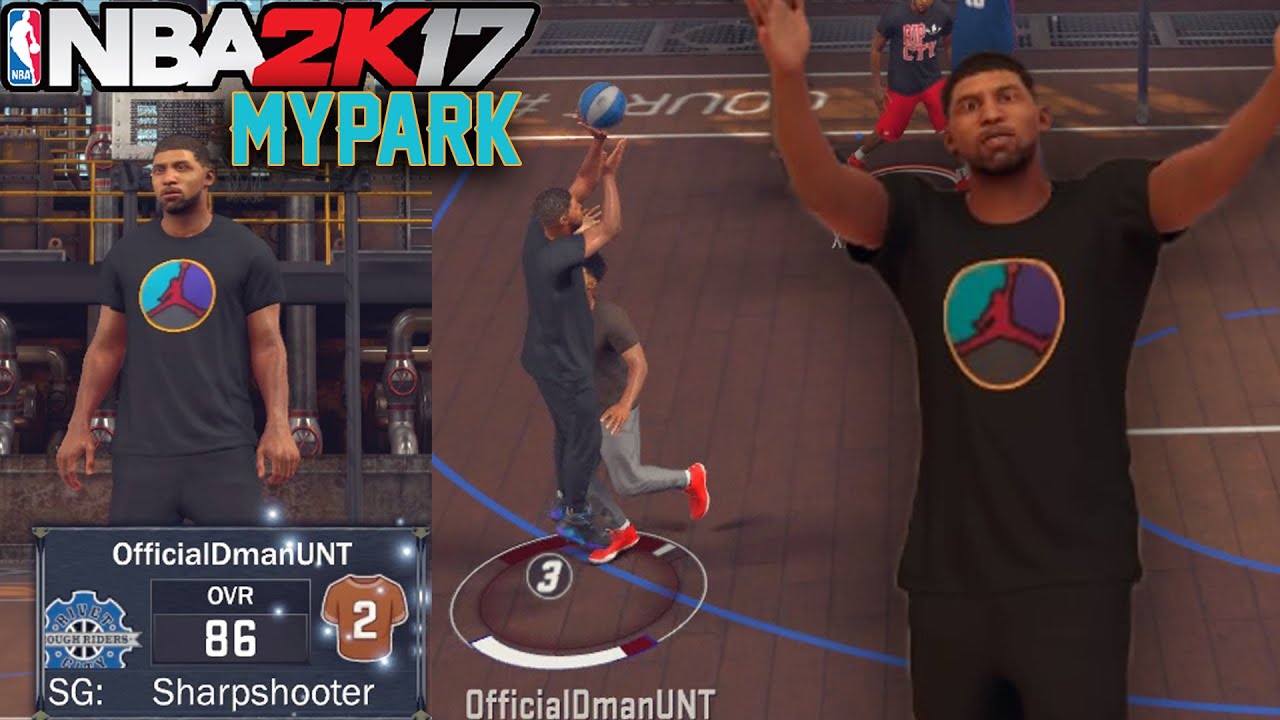Screenshot Caption:  
In this detailed screenshot from the NBA 2K17 video game, the interface highlights the "My Park" mode, identified by the large baby blue lettering across the lower portion of the screen. The iconic NBA logo is prominently displayed in the upper left corner, emphasizing the game's official branding, followed by the "NBA 2K17" title in silver and red fonts.

The highlighted player is identified as "Official D-Man," boasting an impressive overall rating (OVR) of 86. He is classified as an SG (Shooting Guard) Sharpshooter, pointing to his expertise in long-range shots. The character, a black man dressed in a black t-shirt and black shorts, stands against the backdrop of a rundown industrial parkway building, giving a gritty urban feel to the game environment.

On the right-hand side of the screen, we see the character engaged in a gameplay action, shooting from behind the blue three-point line, emphasizing his sharpshooting skills. Adjacent to this is a close-up shot of the player, further showcasing the game's detailed character modeling and customization features.

This screenshot captures the immersive experience of NBA 2K17's My Park mode, where players can create and engage with custom characters in a virtual basketball environment.